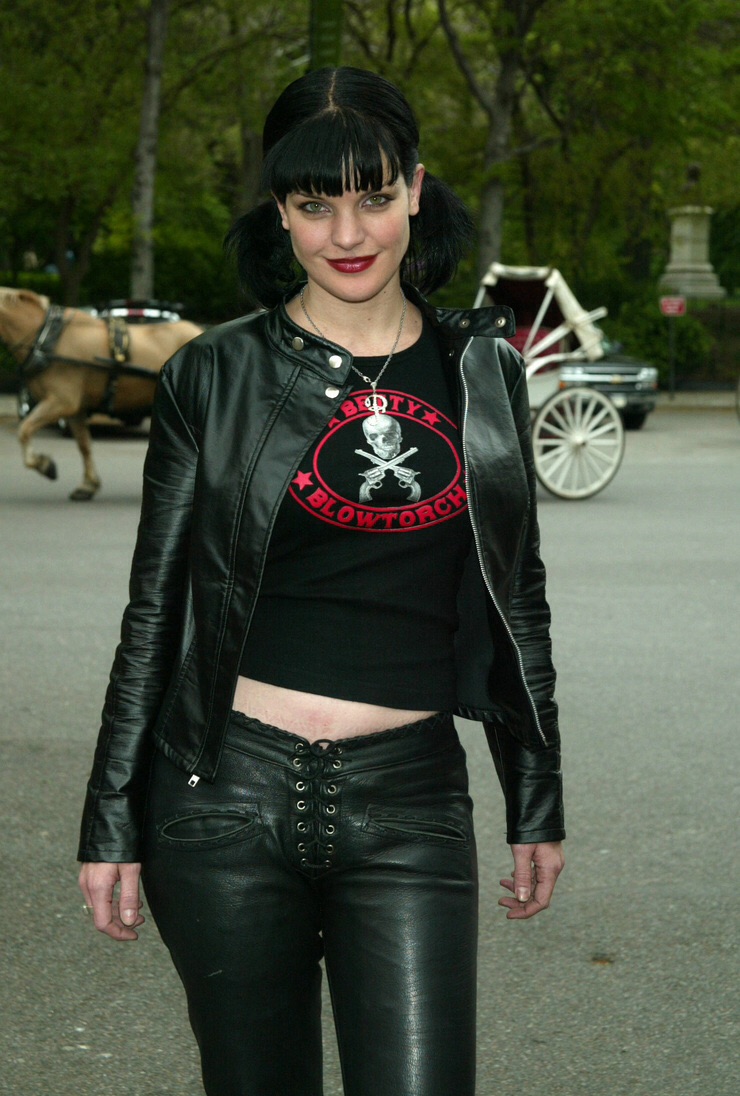In this tall rectangular photograph, a woman poses confidently, visible from the knees up, standing on a gray concrete area likely situated in Central Park, New York. She has pale white skin and dark black hair styled into pigtails with sharp bangs, complemented by striking red lipstick. Her attire is a striking ensemble of black leather: she dons a black leather jacket over a black T-shirt, which features a white skull with crossed guns and the word "Blowtorch" in bright red font, and this T-shirt reveals her belly button. Her fierce look includes black leather pants that lace up where a zipper would typically be and a necklace adorning her neck. She is slightly smirking and gazing directly into the camera.

In the background, to her left, a light brown horse is captured in mid-step, harnessed to a white-wheeled carriage situated on her right. Behind the horse and carriage, there stands a backdrop of tall trees with white and brown trunks and light green leaves. Additionally, in the top right corner, a statue on a white pedestal can be glimpsed through the trees. The scene is vibrant and bustling yet serene, capturing a moment of juxtaposed quiet elegance and urban vigor.